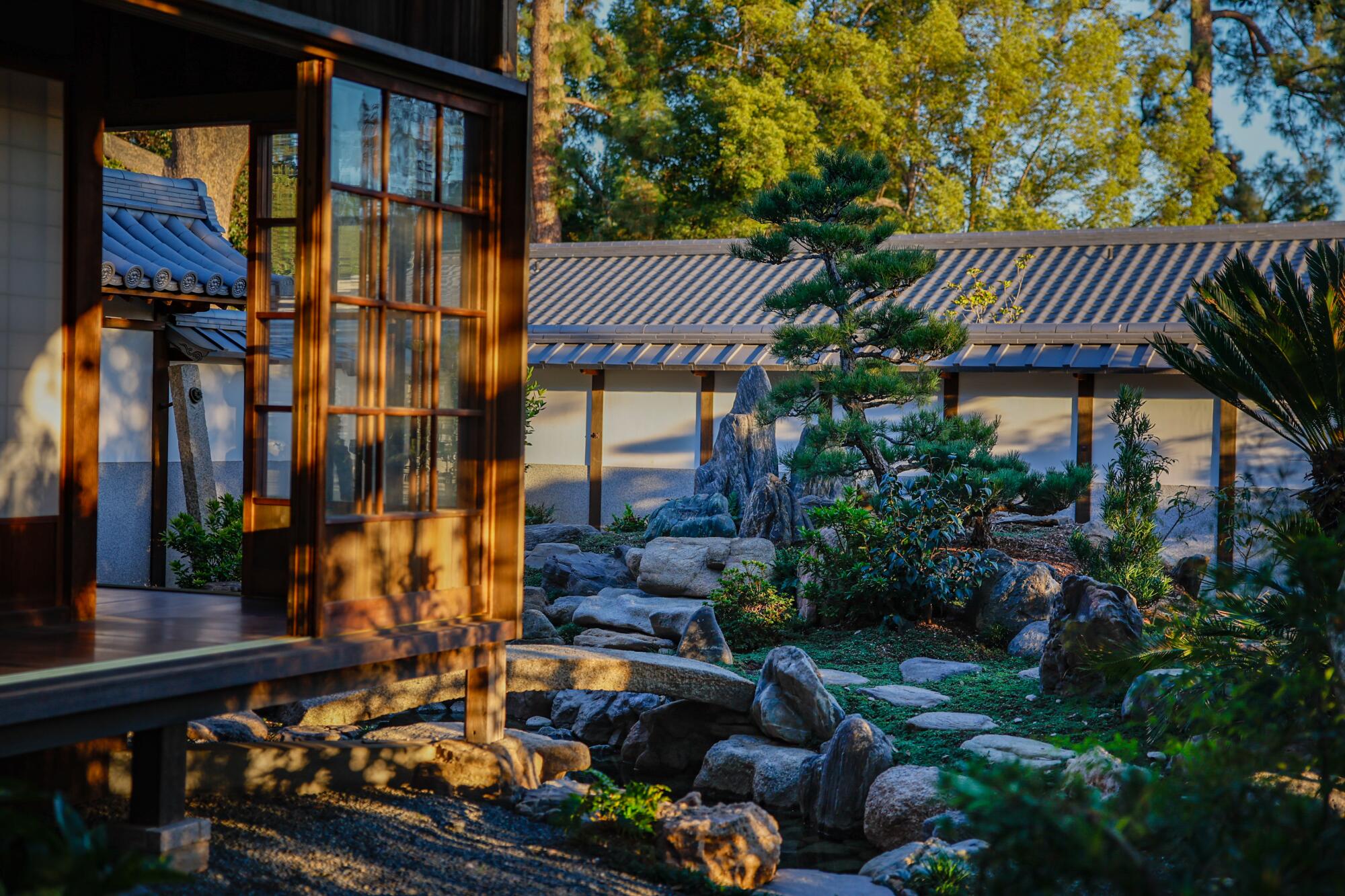This photograph captures a serene Japanese garden scene nestled within a natural and rural setting. The most prominent feature is a pair of traditional Japanese wooden buildings. The nearest building stands on wooden posts set on stone blocks, elevating it above the ground. Its construction includes dark wood and classic shōji paper sliding walls. The second, narrower building at the back also features these traditional paper walls, giving it an elongated greenhouse-like appearance. Both buildings are framed with wood and feature tiled, tilted roofs. 

The garden is meticulously designed with an assortment of greenery, including pine trees, bushes, and vibrant plants. Large stones, stepping stones, and a stone walkway are thoughtfully placed throughout, blending harmoniously with the natural environment. A simple stone arch bridge gracefully spans part of the garden. The setting sun casts a warm, orange light, complemented by a subtle blue hue, suggesting dusk. The overall color palette of the scene is earthy, dominated by greens and browns, creating a tranquil and picturesque atmosphere.